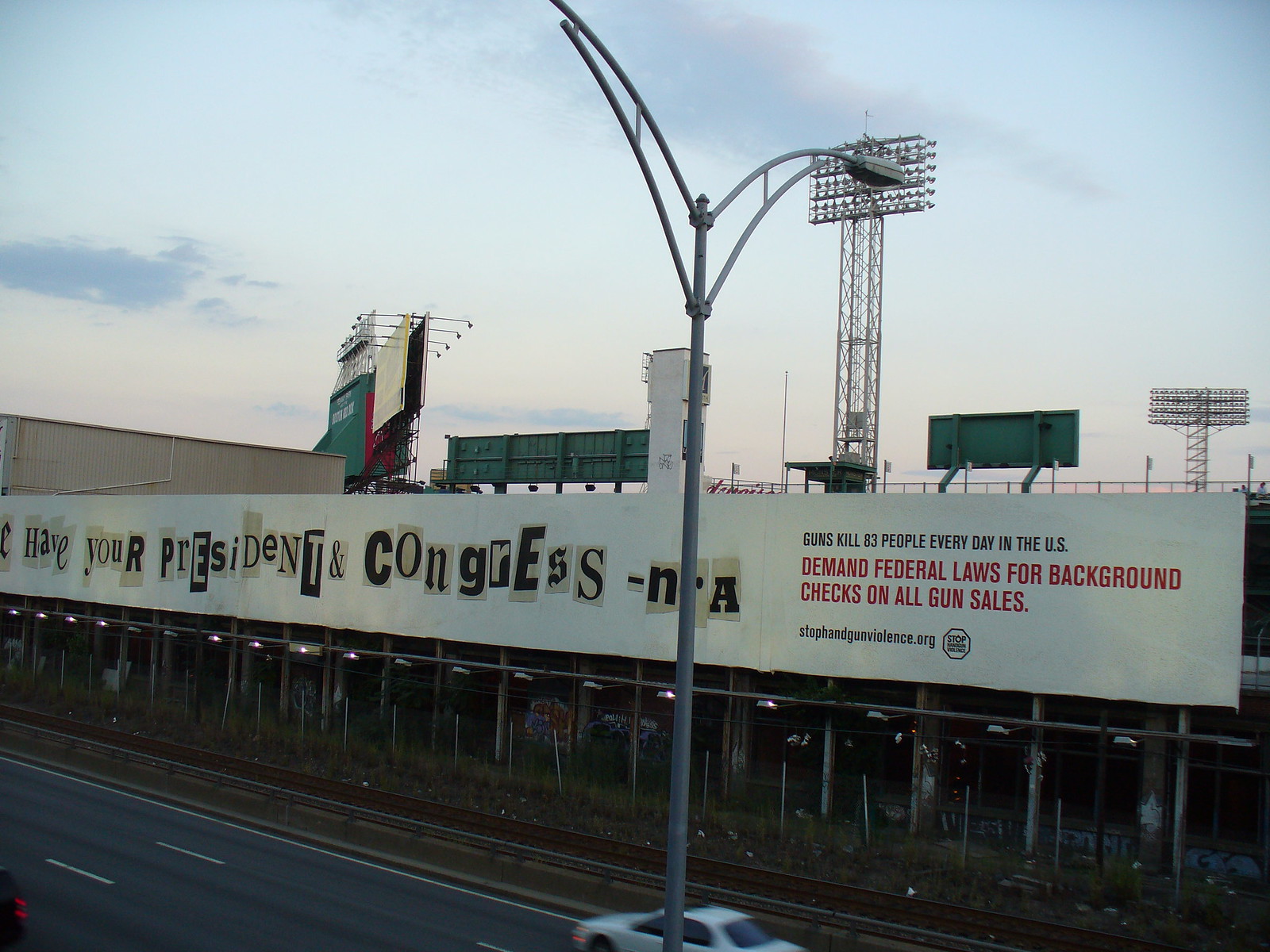The image depicts a large building that closely resembles a stadium, particularly with its architectural design and surrounding elements. In the background, the structure's resemblance to a stadium is further accentuated by the visible backs of billboards and several towering stadium lights. In the foreground, the building prominently features what appears to be the facade of a business establishment. A continuous white-bordered sign spans the length of this side of the structure. On this sign, a partially obscured message reads, "Have your president in Congress - N%A," with the obscured middle letter hidden by a streetlight that extends from the bottom center towards the top center of the image. The combination of these elements creates a puzzling and intriguing scene.